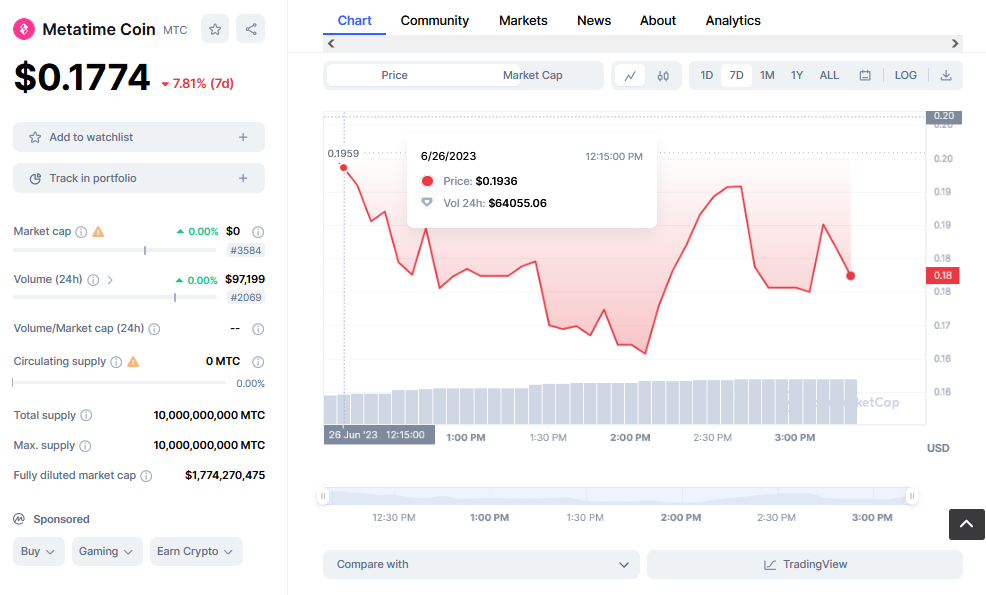The image presents a comprehensive interface showcasing the price action of Metatime Coin (MTC). Dominating the right-hand side is a detailed visual chart that tracks MTC's price fluctuations and trading volume over the past 24 hours. This chart is currently set to display data for a single day but includes adjustable time scales, allowing users to view price trends over 7 days, 1 month, 1 year, or even longer.

At the top of the screen, a navigation bar offers several options, including Chart (the currently selected view), Community, Markets, News, About, and Analytics. This allows users to easily switch between different types of information and resources related to Metatime Coin.

The left-hand side of the interface includes the current price of MTC, along with its percentage change over the past 7 days. Additional options here allow users to add MTC to a watchlist or track it within a portfolio. Other pertinent details displayed include the market capitalization, the trading volume over the last 24 hours, the total supply of MTC, and its maximum supply. This thorough layout provides a holistic view of Metatime Coin's market performance and relevant statistics.